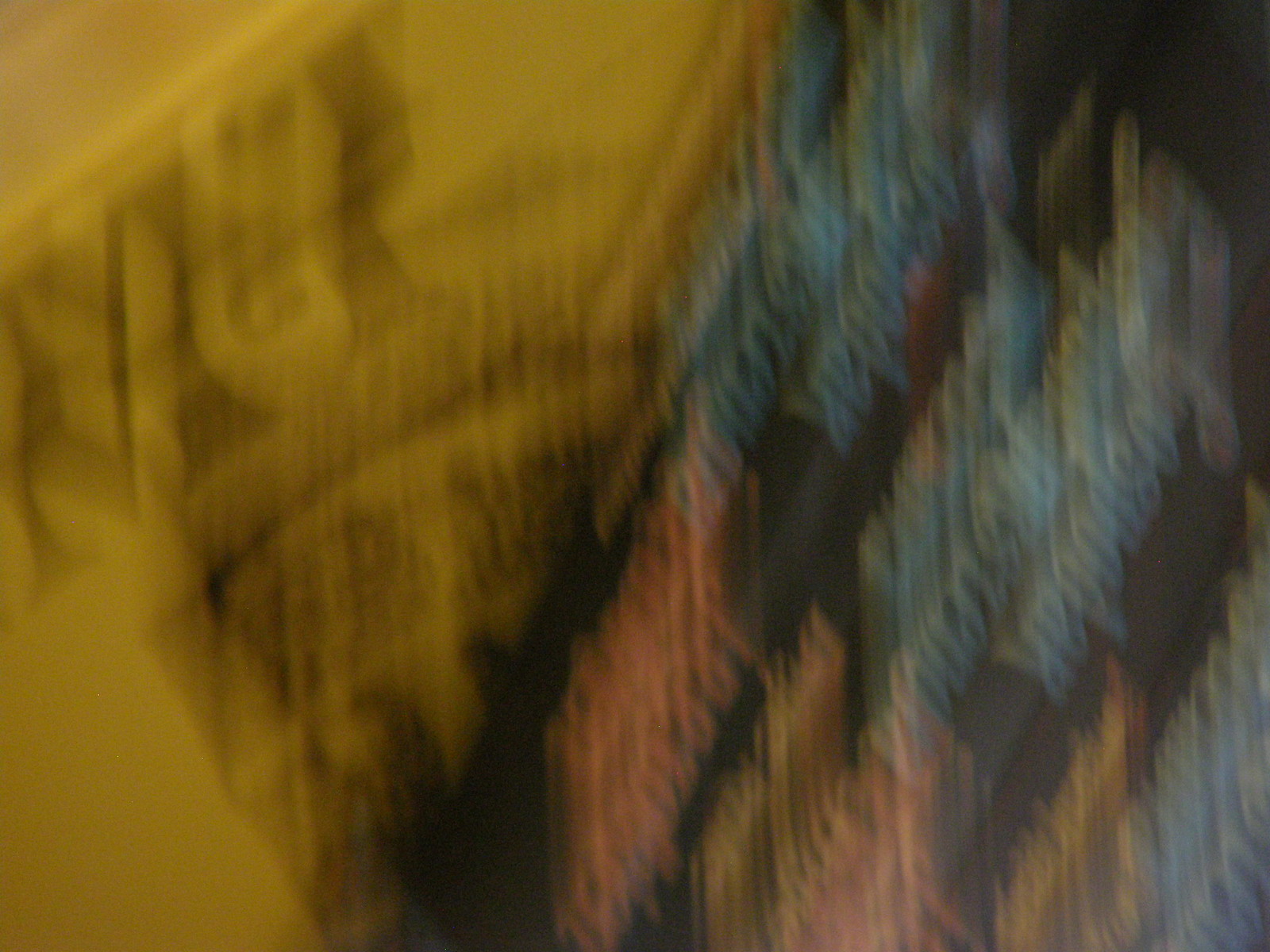This is an extremely blurry photograph where the details are difficult to discern. The composition appears to feature two signs. To the left, there is a yellow sign with black text, possibly indicating a word that begins with "No." The text is written in a script style, and the sign itself seems to be tilted, with the words oriented towards the top left of the image. On the right side, there's a black sign bearing white and pink print, though the specific content of the text remains unclear due to the blurriness of the image. The overall impression is of moving elements within the frame, contributing to the lack of clarity.